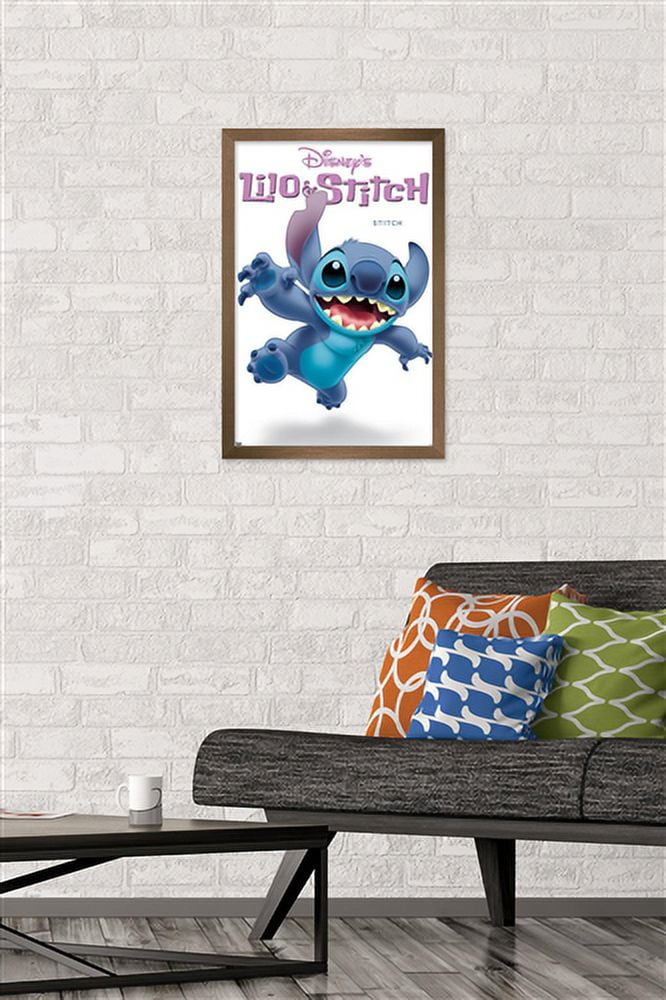The photograph depicts a well-lit living room with a portrait layout. Dominating the backdrop is a white, brick-patterned wall. Central to the wall is a bronze-framed picture featuring Disney's Lilo and Stitch, highlighted by purple lettering at the top and a vibrant image of Stitch in blue, showcasing its claws, pointy teeth, and bulging eyes, as it appears to leap out of the frame. Below the picture, a dark gray and black futon is positioned, adorned with three distinct pillows: a blue pillow with a design, an orange pillow with a circular pattern, and a green pillow. To the lower left of the image, there is a minimalist black coffee table with a white coffee cup placed on it. The floor complementing the modern aesthetic is a charcoal gray wood or laminate finish. The overall setting is bright and clear, emphasizing the vivid details and cozy ambiance of the living room.